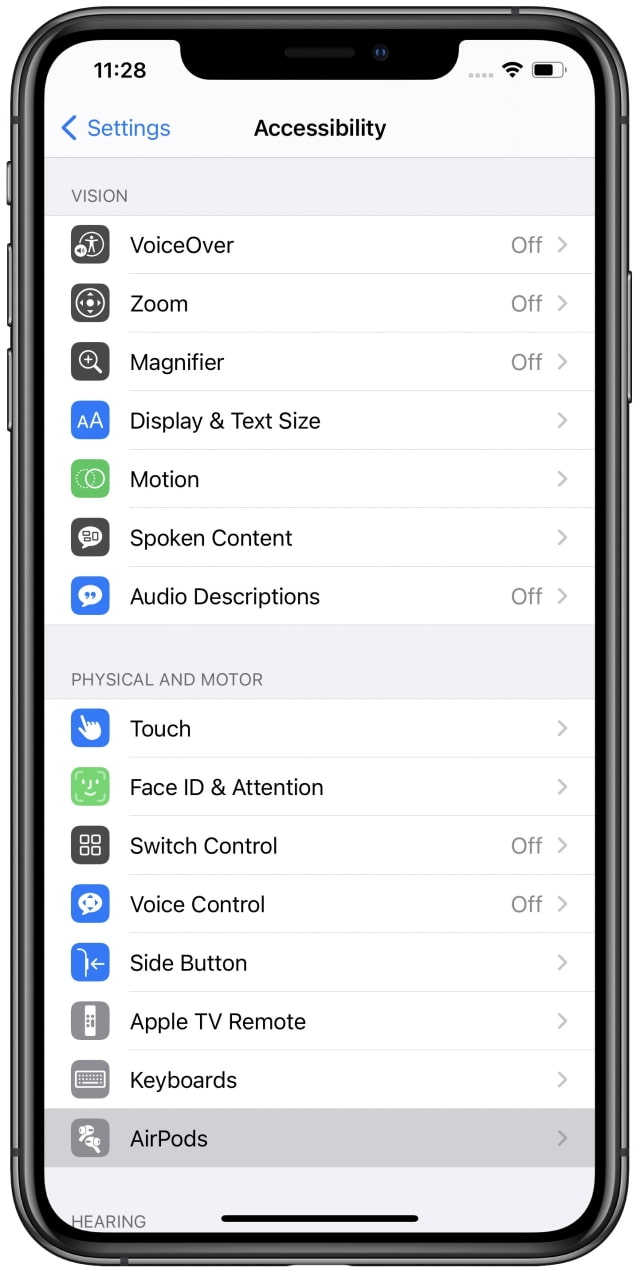**Detailed Caption:**

This image showcases the Accessibility settings screen on an iPhone, captured at 11:28 AM with a strong Wi-Fi connection and approximately 75-80% battery life. At the top, "Accessibility" is prominently displayed, indicating the focus of the settings. The settings are categorized and visually represented with icons next to each subheading. 

Under the "Vision" category:
- **VoiceOver**: Displayed off, represented by a gray icon of a person within a circle and a sound wave.
- **Zoom**: Off, indicated by directional arrows (north, south, east, west) within a circle.
- **Magnifier**: Off, marked by a magnifying glass with a plus sign inside.

In the "Display & Text Size" section:
- **Display & Text Size**: Noted with a blue icon featuring white writing.
- **Motion**: Represented by two entwined circles on a green background.

For "Spoken Content" and "Audio Descriptions":
- **Spoken Content**: Depicted with a speech bubble icon containing shapes.
- **Audio Descriptions**: Shown with a speech bubble enclosing quotation marks.

Within "Physical & Motor":
- **Touch**: Illustrated by a finger pointing icon.
- **Face ID & Attention**: Represented by a face with a broken square.
- **Switch Control**: Displaying four small squares within a larger square.
- **Voice Control**: Indicates with directional arrows (north, south, east, west) inside a speech bubble.
- **Side Button**: An arrow points to the button on a side of the phone.
- **Apple TV Remote**: Shows a small image of the remote.
- **Keyboards**: Represented by an icon of a keyboard.
- **AirPods**: Depicted with icons of AirPods.

At the bottom of the screen, the next category "Hearing" is partially visible, suggesting more settings below. Each icon's color scheme and design provide a visual aid to differentiate between the various accessibility features available on the iPhone.